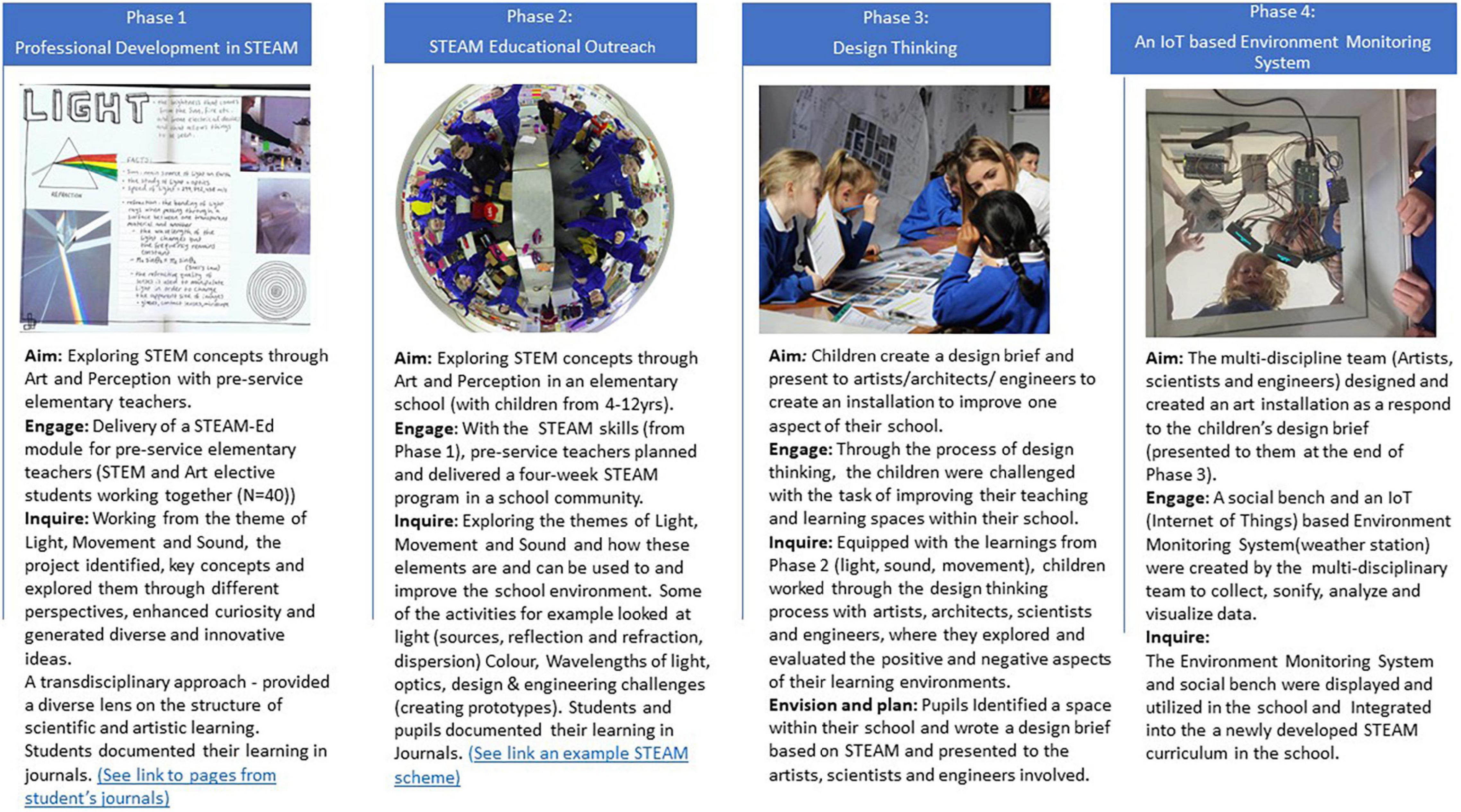This informational poster consists of four distinct columns on a white background, each demarcated by a blue border at the top indicating the various phases of a STEAM-focused program. 

- **Phase 1: Professional Development in STEAM** - Aims to explore STEM concepts through art and perception specifically with pre-service elementary teachers. It features a paper illustrating light reflection. The objective includes engaging delivery of STEM education modules and encouraging collaboration among 40 STEM and art elective students. This phase investigates key concepts like light, movement, and sound, promoting curiosity and innovative ideas via a transdisciplinary approach. Students documented their insights in journals, accessible through a provided link.

- **Phase 2: STEM Educational Outreach** - Accompanying this section is a mirrored round image of children collaborating around a table in a classroom setting. This phase focuses on extending STEM education beyond the initial group, emphasizing broader community engagement.

- **Phase 3: Design Thinking** - Depicts students and teachers collaboratively working on a design project. This phase is centered on iterative problem-solving and creative ideation, guiding participants through the process of coming up with solutions and creating prototypes.

- **Phase 4: IoT-based Environment Monitoring System** - Shows a practical application scene where students are involved in assembling a product, complete with wires and batteries. This represents the application of learned concepts in real-world scenarios, focusing on the integration of Internet of Things (IoT) technologies for environmental monitoring.

Each column provides detailed descriptions of the aims, design, and inquiry questions pertinent to the respective phases, offering a comprehensive overview of the multi-faceted approach to STEAM education articulated in the program.